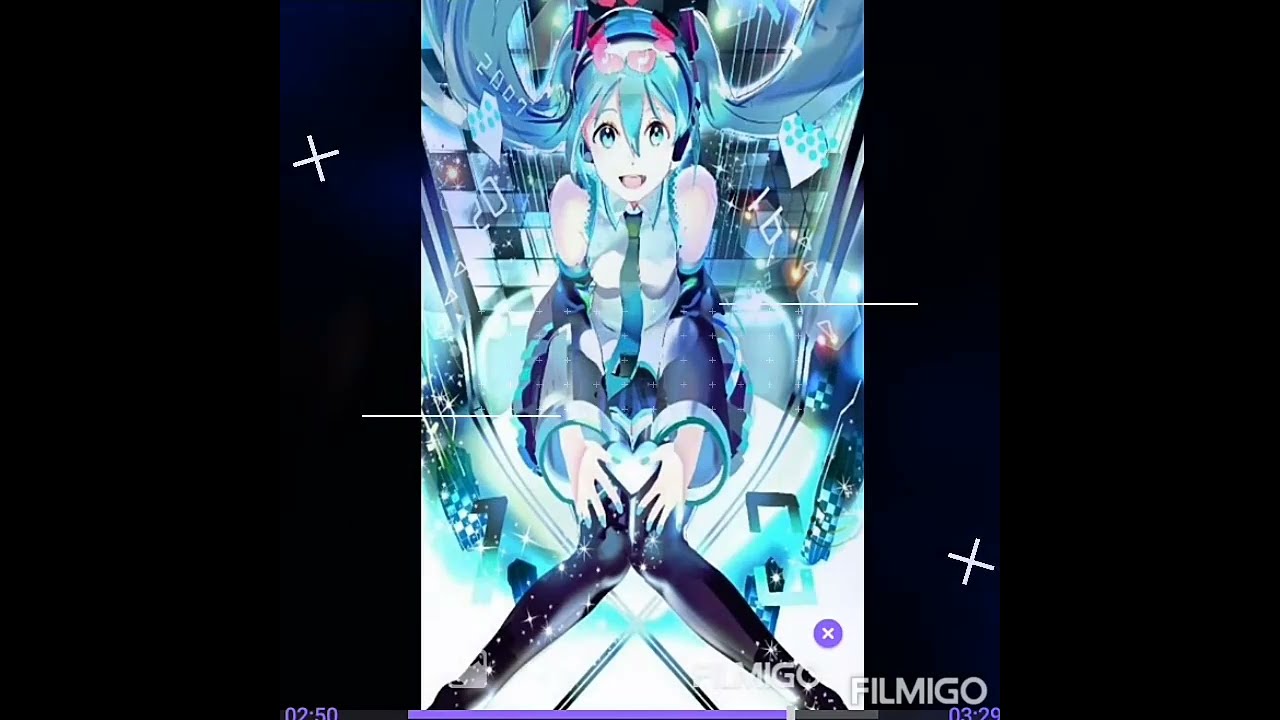This image is a detailed and vibrant depiction of a female anime character, likely from a video game or anime cartoon. The central figure, a young girl with blue hair and big blue eyes, exudes a charming and welcoming aura with her open-mouthed smile. Her attire is a blend of blue and white hues, consisting of a light blue sleeveless shirt paired with a dark blue tie, and complemented by dark-colored stockings. Her bare shoulders lead to long blue sleeves that start from the elbows, tied with ribbons. Positioned with her knees together and hands resting on her thighs, she sits serenely, possibly on a heart-shaped object surrounded by a blue ring.

The background enhances the overall blue theme, featuring shiny glass figures and a black and white square tile pattern that adds depth and contrast. On the bottom right corner, there is a watermark that reads "Fill me go." The image is framed by two thick vertical black strips on the left and right sides, the left strip adorned with a white plus sign, giving it a letterbox appearance. This framing emphasizes the central composition of the character, highlighting her serene and joyful expression amidst a dynamic and visually appealing setting.